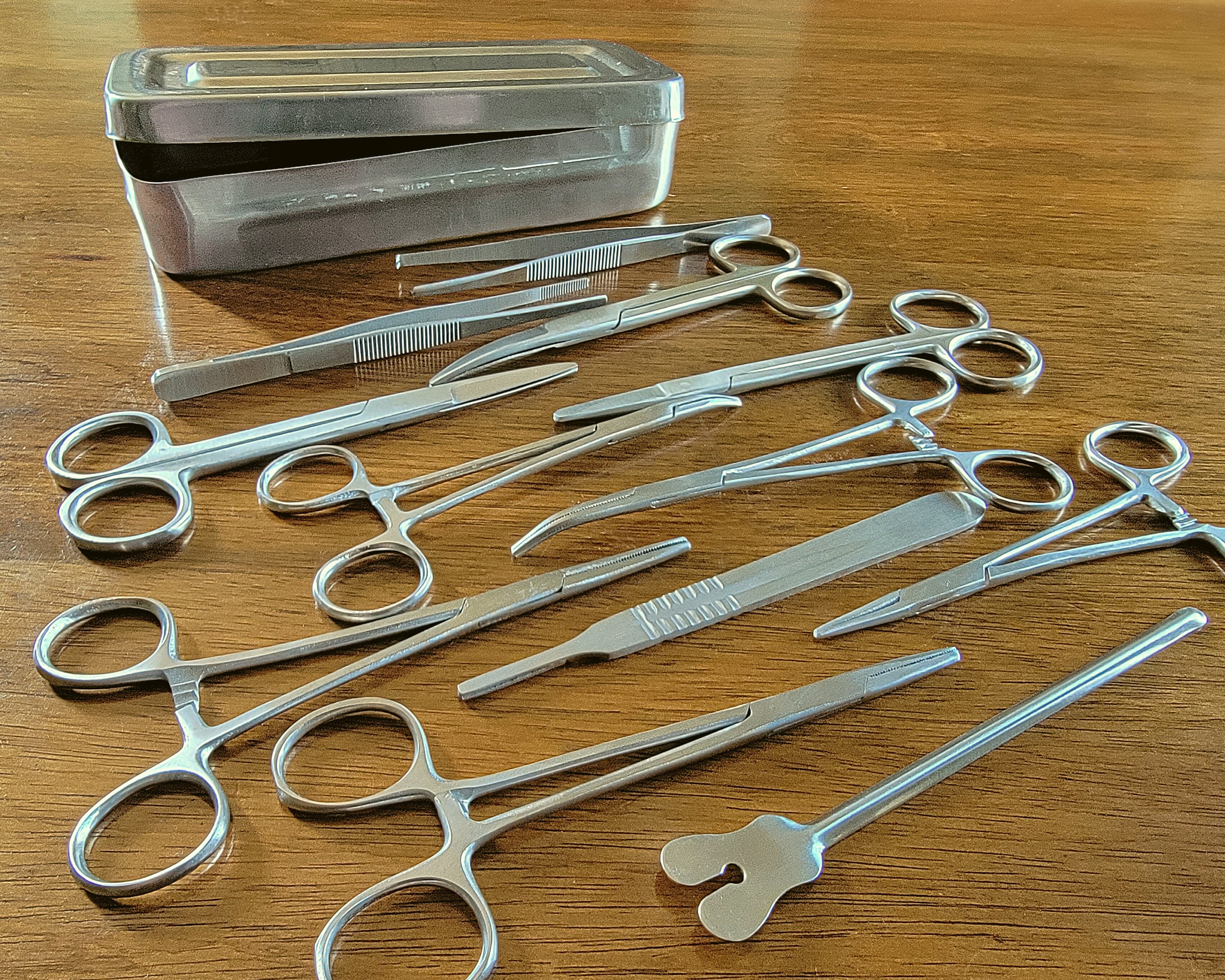A collection of vintage-looking medical instruments is meticulously arranged on a wooden surface. The set includes a retractor, various types of tweezers (both straight and curved), different forceps, and numerous scissors, some with bent tips. The instruments, numbering twelve in total, show signs of use with visible scrapes and wear and are primarily locking instruments with some having intricate locking mechanisms on the handles. The items are aligned in two groups, with each group facing inward, their sharp ends pointed towards each other. In the background, a slightly ajar metal pan, potentially used for storing or sterilizing these tools, completes the scene. The entire setup hints at a potential sale display or an organized collection, showcasing the polished, stainless-steel instruments in a contrasting wood grain backdrop.